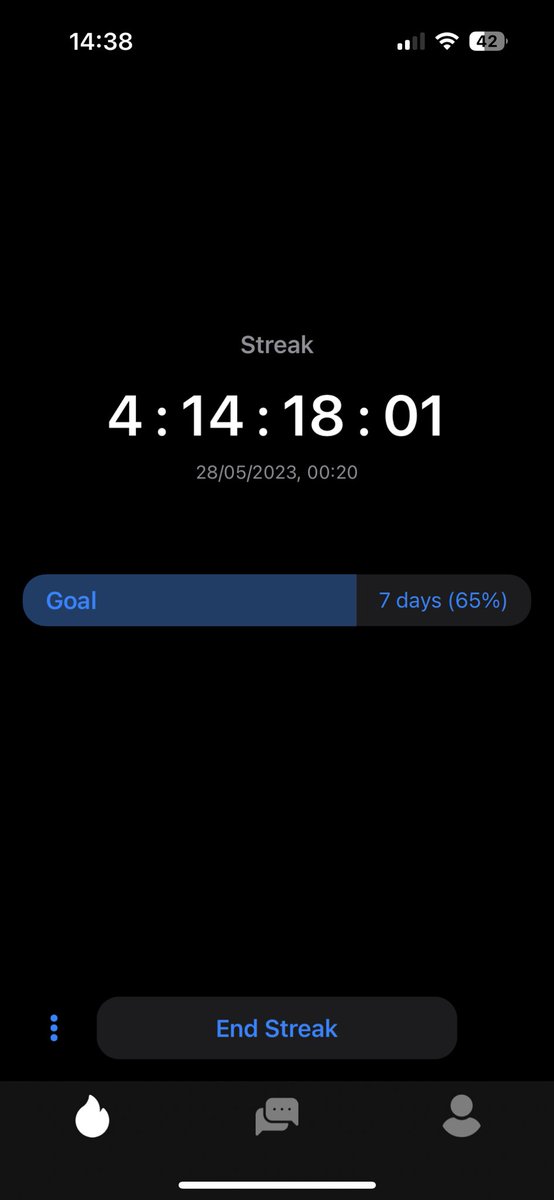This screenshot captures a detailed view of a timekeeping application on a smartphone. The screen has a sleek black background along the top where, on the left, the current time is displayed as "14:38." To the right, there are signal indicators showcasing four bars, with only two bars illuminated, followed by a Wi-Fi icon and a battery icon displaying "42%" charge remaining.

Centered on the screen, the word "Streak" is prominently displayed. Directly beneath it, a timer reads "04:14:18:01," indicating a countdown or elapsed time in days, hours, minutes, and seconds. Below the timer, in smaller text, the date "28-05-2023, 00:20" is shown, possibly denoting the start time or a significant timestamp.

A blue progress bar spans the width of the screen beneath the date. The bar is rounded at both ends, with the text "Goal" occupying the left two-thirds and "7 days, 65%" on the right, indicating the user's progress towards a weekly goal.

At the bottom of the screen, a dedicated section in blue text invites the user to "End Streak." Below this, there is a navigation bar divided into three sections, each featuring a distinct icon to represent different functions or sections within the app.